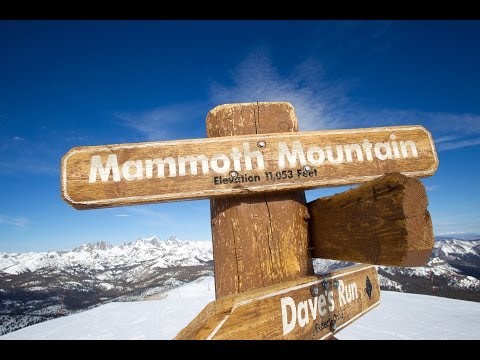The image is a rectangular photograph, wider than it is tall, bordered with a thin black line. Dominating the background, a broad expanse of dark blue sky gradually lightens towards the horizon, with wispy clouds scattered throughout. Below the sky, a rugged mountain range stretches across the scene, its peaks and ridges covered in snow. 

In the center of the image stands a weathered wooden post with three signs mounted on it. The top sign, with slightly rounded edges, reads "Mammoth Mountain" in bold white letters, noting an elevation of 11,053 feet. Below this, another sign is affixed but only its back is visible, facing to the right, obscuring its text from view. The bottom sign, shaped like an arrow pointing to the left and also topped with a thin white border, reads "Dave's Run."

The focus of the image is the signpost, set against the dramatic backdrop of snow-capped mountains and an expansive sky, indicating that the setting is at or near the summit of Mammoth Mountain. The colors in the scene are dominated by blues, whites, browns, and grays, highlighting the stark, natural beauty of the mountainous landscape.